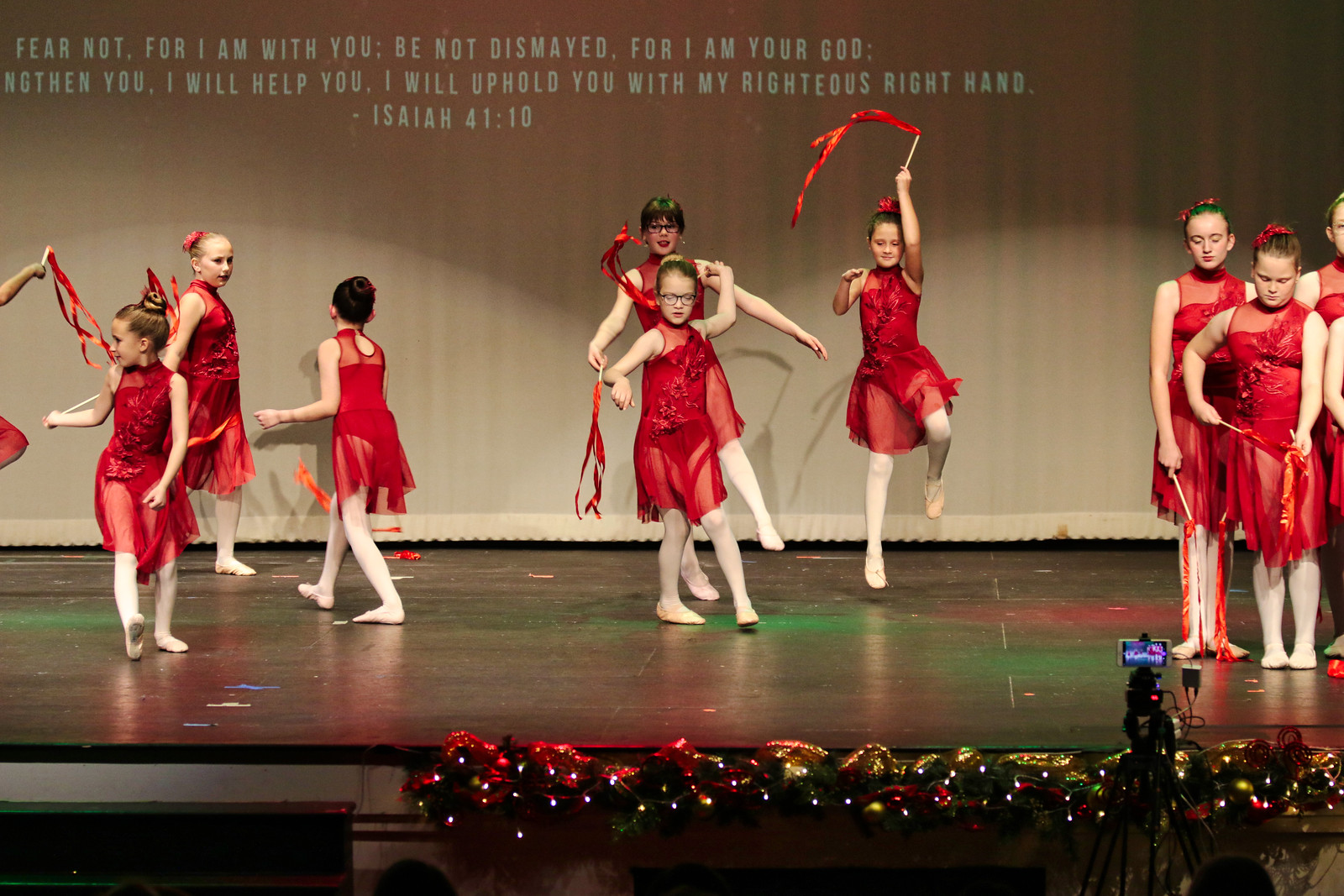The image depicts a festive dance recital at a church, featuring a group of young girls aged around 6 to 12, performing on a stage. They are dressed uniformly in red dresses with solid red leotards underneath and tulle overlays adorned with decorative floral patterns. Each girl wears a red ribbon in her hair, white tights, and traditional pink ballet slippers. They hold sticks with red ribbons attached, gracefully dancing across the stage. The stage is decorated with wreaths, Christmas lights, and ribbons, evoking a holiday ambiance. A camera is positioned at the bottom right corner, capturing the performance. On the back wall of the stage, a biblical verse is projected: "Fear not, for I am with you. Be not dismayed, for I am your God. I will strengthen you, I will help you, I will uphold you with my righteous right hand. Isaiah 41:10." The colors in the scene include shades of red, lighter red, beige, tan, green, blue, and white.